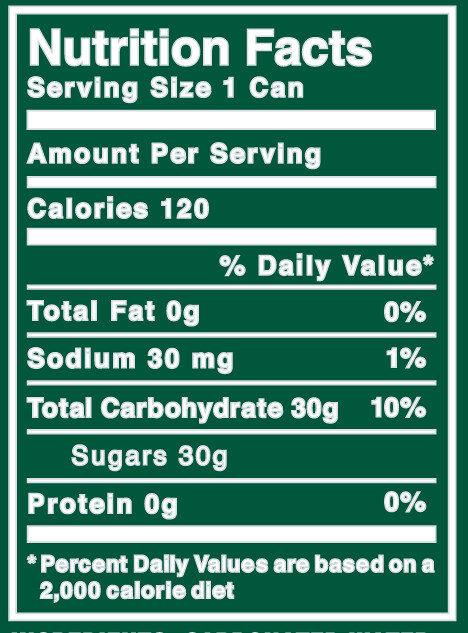The image displays a green vertically-oriented rectangular label with the heading "Nutrition Facts" in white letters. The label indicates that the serving size is one can, and provides nutritional information for a single serving. Key details include:

- Calories: 120
- Total Fat: 0 grams (0%)
- Sodium: 30 milligrams (1%)
- Total Carbohydrate: 30 grams (10%)
- Sugars: 30 grams
- Protein: 0 grams (0%)

Additionally, there is a note at the bottom stating that the percent daily values (%DV) are based on a 2,000 calorie diet, highlighted with an asterisk.